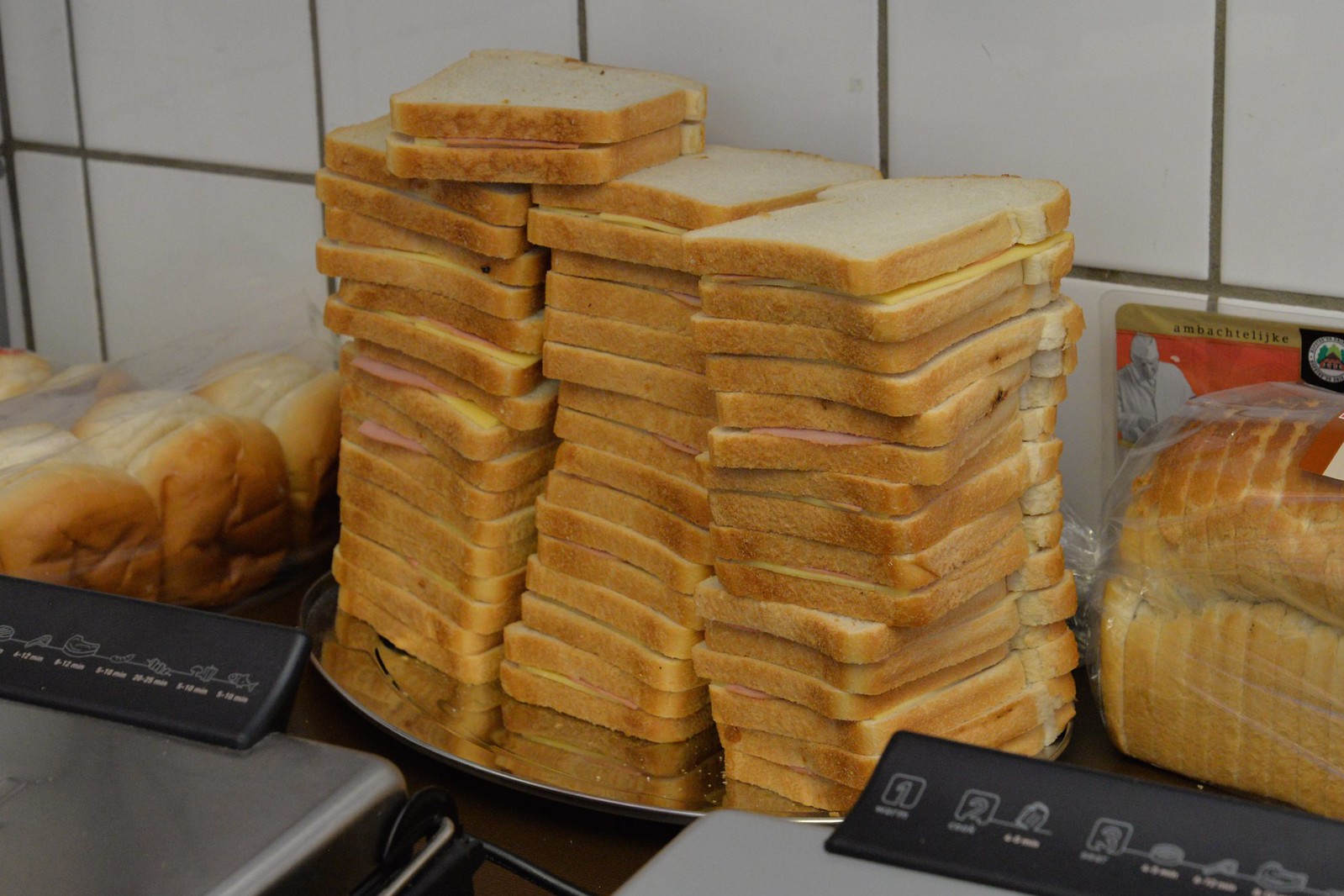The photograph depicts a commercial kitchen environment, featuring a white ceramic tiled wall with dark grey grout. In the center of this setup, three uneven stacks of white bread sandwiches, filled with slices of cheese and deli meat, are arranged on a highly reflective silver oval platter. To the left, a clear plastic bag contains hamburger buns, while an additional pre-packaged loaf of white bread is partially visible on the right. The setting includes stovetops on both sides of the counter; their control panels are black plastic with various illegible symbols, hinting at the appliances' functional purpose. The overall scene suggests a high-volume sandwich preparation, possibly for a restaurant or catering service.